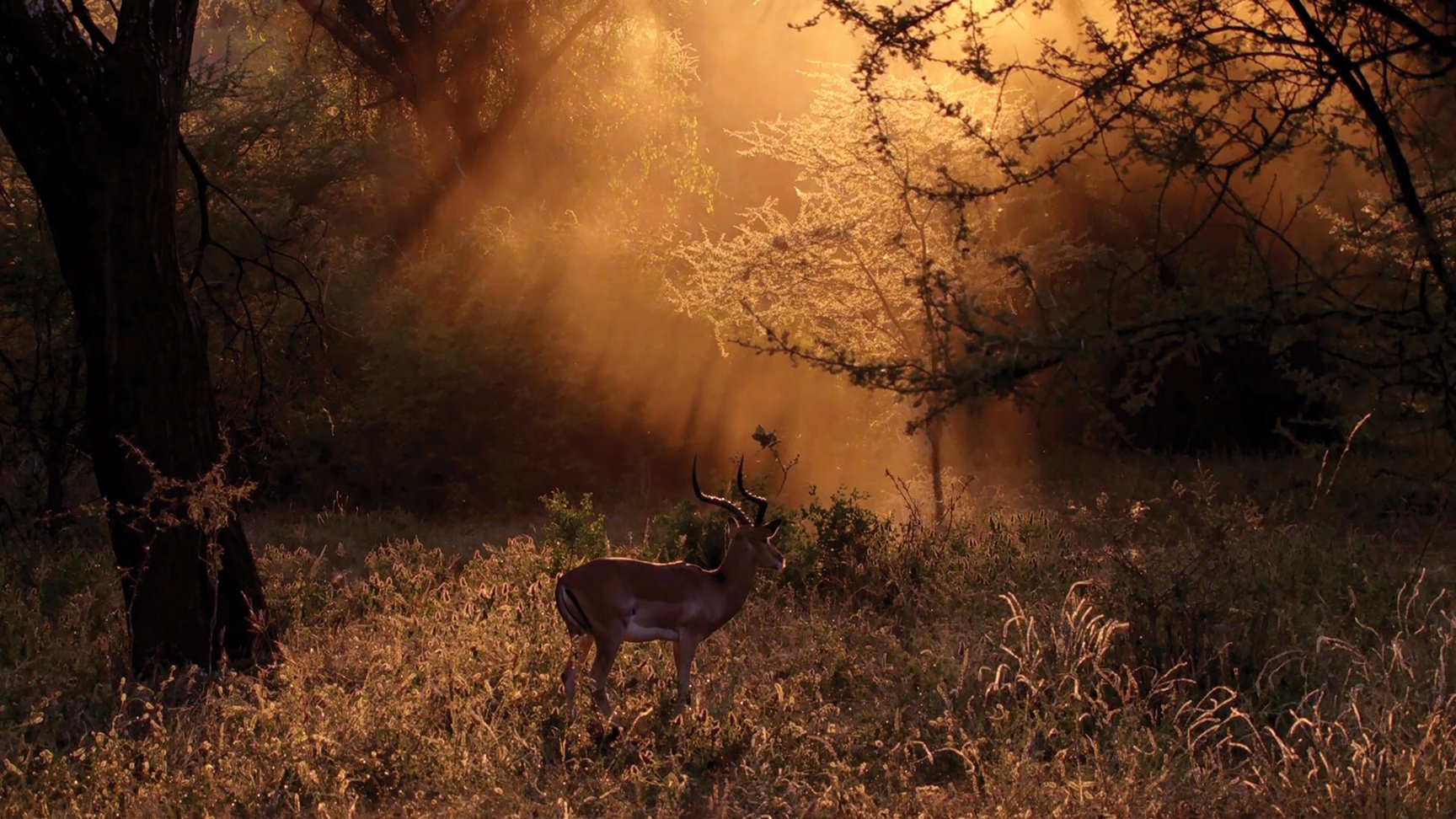The image is a detailed and moody painting of a dense forest landscape bathed in a sepia-toned glow. Lush yet brownish-yellow grass carpets the ground, and a heavenly light shines through the fog, casting a mystical aura over the scene. In the center of the painting stands a majestic deer, possibly a gazelle or an antelope, with beautifully curved horns. The deer, illuminated by the light breaking through the canopy, appears cautious, staring off to the right amidst the misty surroundings. Large tree trunks, both illuminated and shadowed, frame the composition, with particularly notable dark dead trees on either side. The combination of the fog, the play of light and shadow, and the intricate detailing of the foliage and the deer itself, imbues the image with an ethereal early-morning atmosphere.